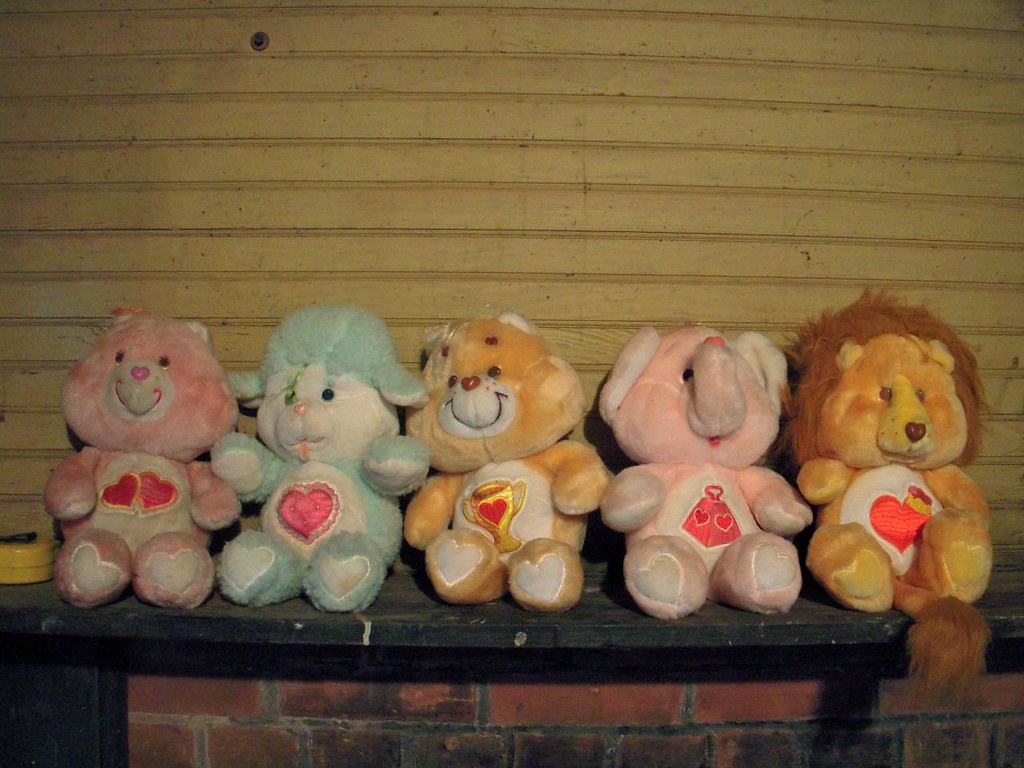The image depicts five stuffed animals, resembling vintage Care Bears, seated on a narrow, black mantel above a red brick fireplace. They are displayed against a backdrop of horizontally arranged wooden slats. From left to right, the lineup includes a pink and white bear bearing two hearts on its belly, a blue and white sheep with a single heart, an orange-ish brown bear featuring a gold trophy with a heart in the center, a pink and white elephant with a long trunk and a triangle emblem, and a brown, orange and white lion with a bushy mane and a heart symbol. These carefully arranged stuffed animals add a nostalgic charm to the rustic setting.